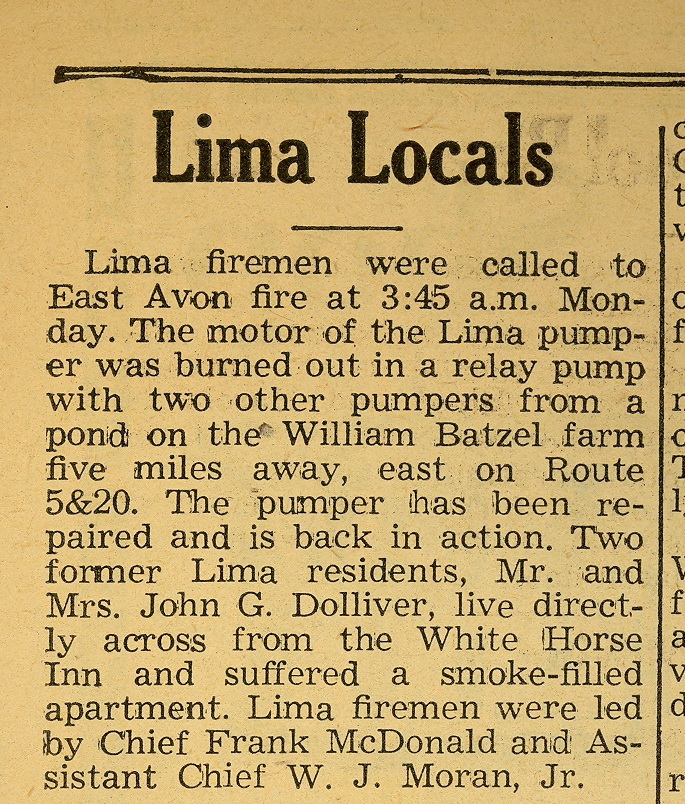This image depicts an old newspaper article section titled "Lima Locals" in large black font on a beige, aged paper. Beneath the title, a thin horizontal black line separates it from the main body of text. The article reports that Lima firemen were called to a fire in East Avon at 3:45 a.m. on Monday. During the incident, the motor of the Lima pumper was burned out while relaying with two other pumpers from a pond located on the William Betzel Farm, five miles east on Route 5 and 20. It notes that the pumper has since been repaired and is back in service. The article also mentions that two former Lima residents, Mr. and Mrs. John G. Dolliver, who lived directly across from the White Horse Inn, experienced a smoke-filled apartment. The firefighting team was led by Chief Frank McDonald and Assistant Chief W.J.W. Moran, Jr. Additionally, a vertical black line runs down the right side of the article, indicating the presence of adjoining paragraphs, with the first letters of these subsequent lines barely visible at the edge of the clipping.